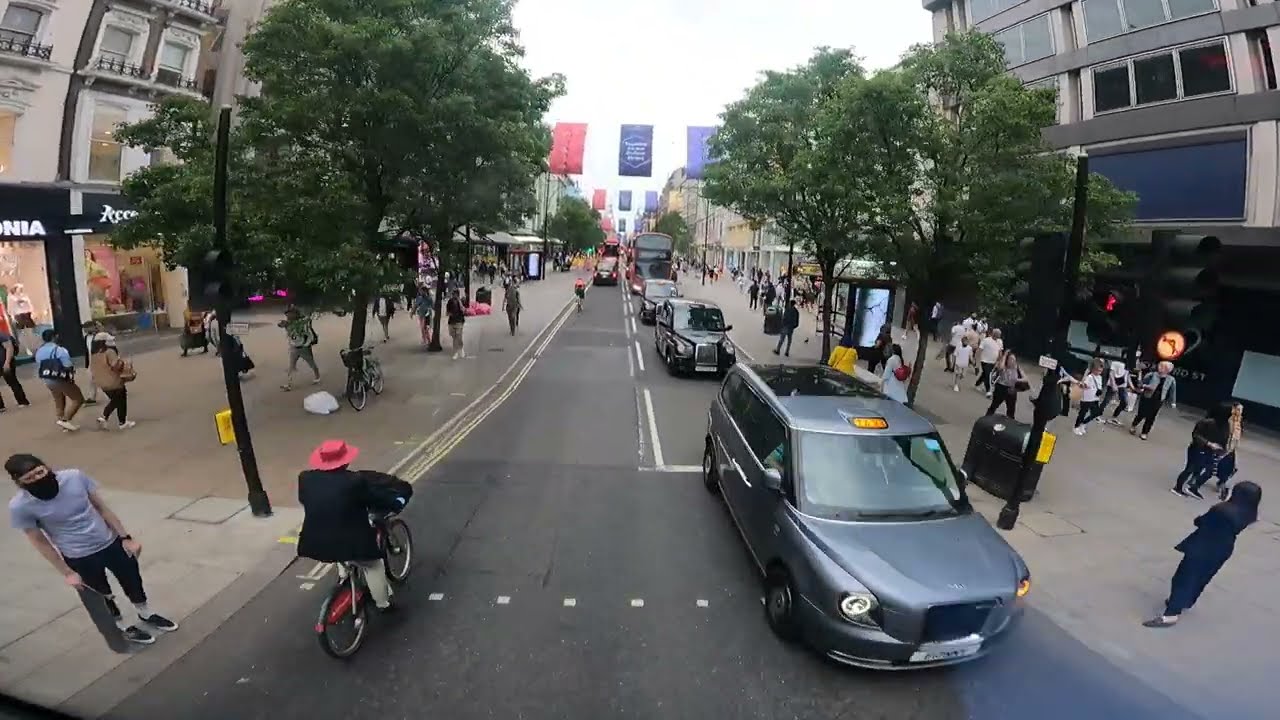This photograph captures a bustling city street, also known as a C-Street, lined with trees and buildings on either side. The scene is busy with various activities: people walking to and fro on the large sidewalks, bicyclists riding in different directions, and a mix of cars moving both towards and away from the viewer. 

In the foreground, on the lower left-hand corner, there is a man with a skateboard wearing a black mask. Next to him, a person in a black jacket and pink hat rides a bicycle. A gray car is visible near the lower right-hand corner, while a silver car with a white license plate leads a line of vehicles in one lane. In front of it is what appears to be a black car with a silver, squarish grille, followed by a red double-decker tour bus. 

Further up the street, more bicycles can be seen as well as some buses, possibly near shelters. Banners hang across the street halfway up, contributing to the street's festive atmosphere. 

Storefronts with large windows and black awnings can be observed on the left side, while a significant building stands on the right. The road has white markings and appears a bit wobbly in the middle. Traffic lights and long black vertical posts line the sidewalks, which are also dotted with lamp posts. 

Overall, the image conveys a lively and active urban environment with a variety of movement and architectural details.